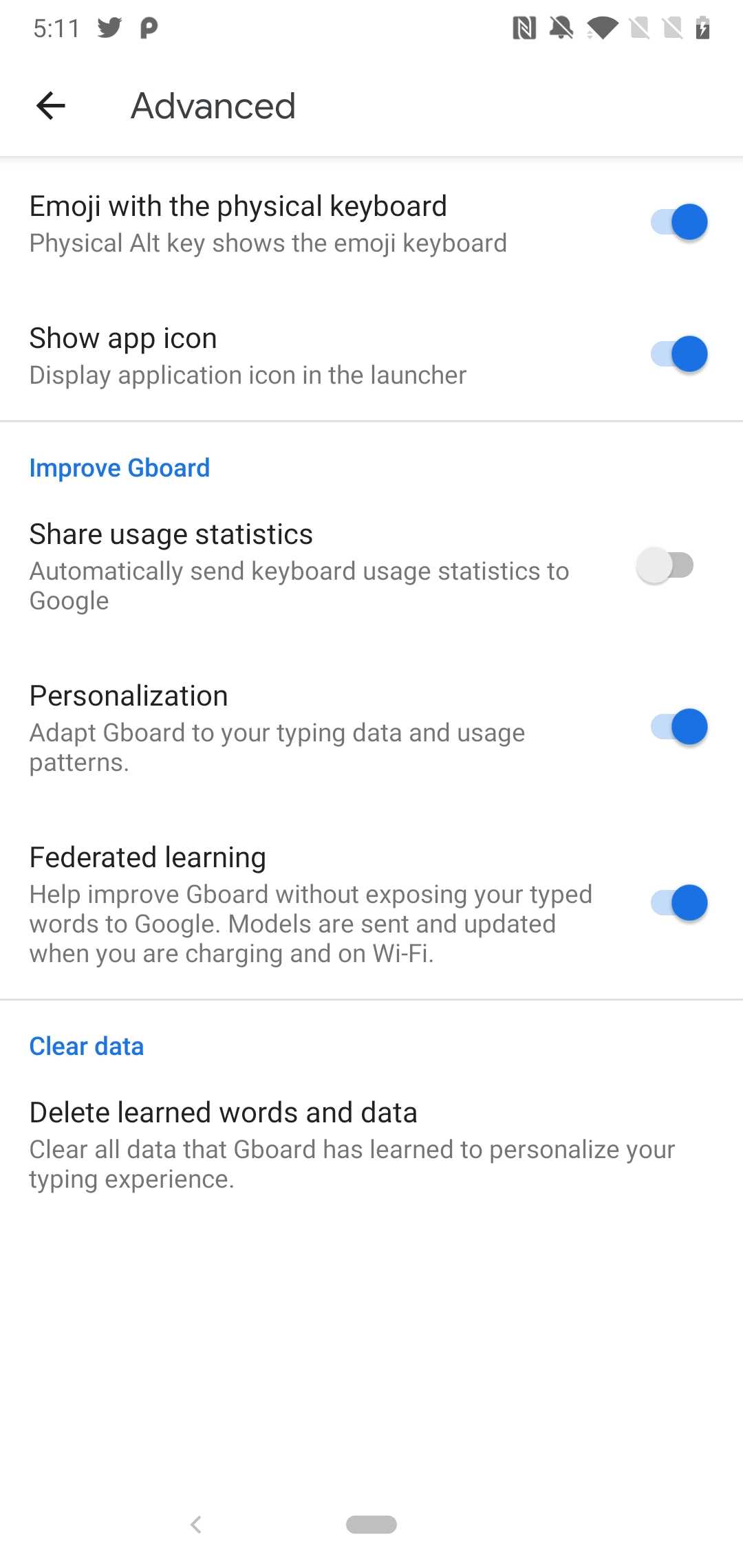The image displays a smartphone screen featuring various settings for the Gboard app. At the very top of the screen are indicators including the time, a Twitter icon, a muted notification bell icon, and battery percentage. 

The main page of the screen has a white background with black text, beginning with a black back arrow that leads back to the previous page. The heading reads "Advanced." 

Following this, the first section labeled "Emoji with a Physical Keyboard" states: "Double Alt Key shows the Emoji Keyboard." This setting is turned on, as indicated by a blue switch.

The next option, "Show App Icon," is described as "Display Application Icon in the Launcher," and this is also toggled on with a blue indicator.

Further down, the "Improved Gboard" section has a setting for "Share Usage Statistics." This states: "Automatically Send Keyboard Usage Statistics to Google," which is toggled off with a gray indicator.

Next in line is the "Personalization" section, stating: "Adapt Keyboard to Your Typing Data and Usage Patterns." This setting is turned on, indicated by a blue switch.

The "Federated Learning" section aims to "Help Improve Gboard Without Exposing Your Typed Words to Google. Models are sent and updated when you are charging and on Wi-Fi." This feature is also activated, as shown by a blue logo.

At the bottom of the screen is the option to "Clear Data," highlighted in blue, suggesting it is clickable. The accompanying description reads: "Deleted Learned Words and Data. Clear all data that Gboard has learned to personalize your typing experience."

Additionally, the bottom of the page features a small gray arrow and a gray icon, completing the screen view.